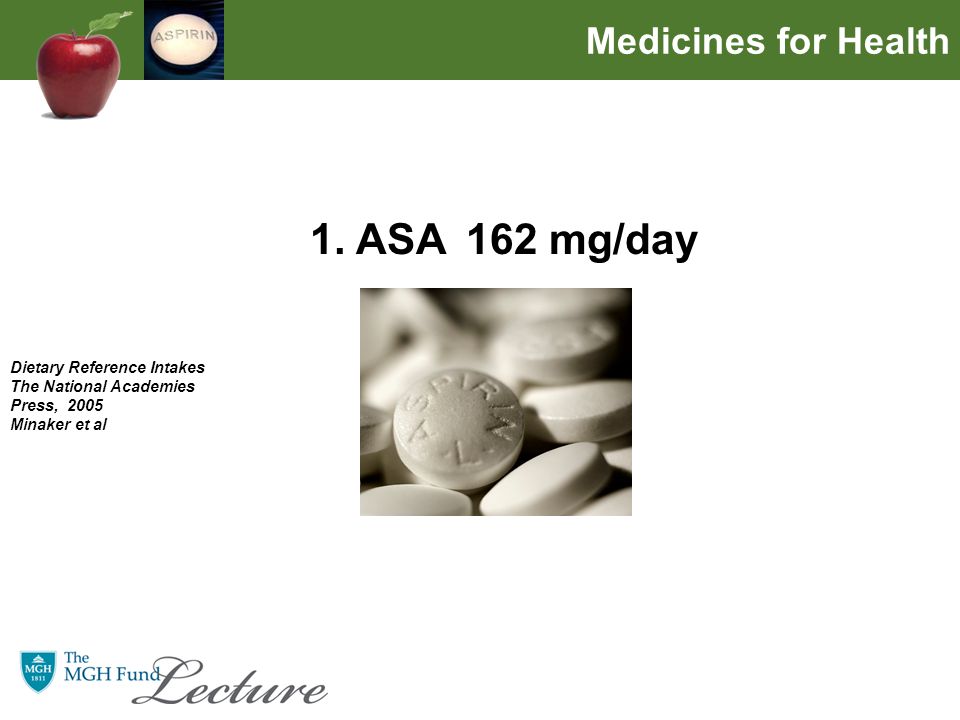The slide appears to be an informational graphic, likely from a PowerPoint presentation, designed to provide detailed information about aspirin. The background is predominantly white, giving the slide a clean and professional look. 

At the top of the slide, a green banner stretches from the left to the right. On the left side of this banner is a red apple with a green leaf, situated next to a square that displays a single circular pill with the word "aspirin" carved into it. On the right side of the banner, white text reads "Medicines for Health."

In the central section of the slide, a black and white photograph features a small pile of round pills, each stamped with the word "aspirin." Above this photograph, bold text states "1. ASA, 162 milligrams/day." To the left of the image, in small black text, it reads "Dietary Reference Intakes, The National Academies Press, 2005, Minsker et al." The bottom left of the slide includes additional text, indicating it is related to "The MGH Fund Lecture."

The overall color scheme includes red, green, black, and white, with occasional blue elements, contributing to the slide's visually informative nature. The design and arrangement of elements aim to effectively communicate information about aspirin usage and its health implications.